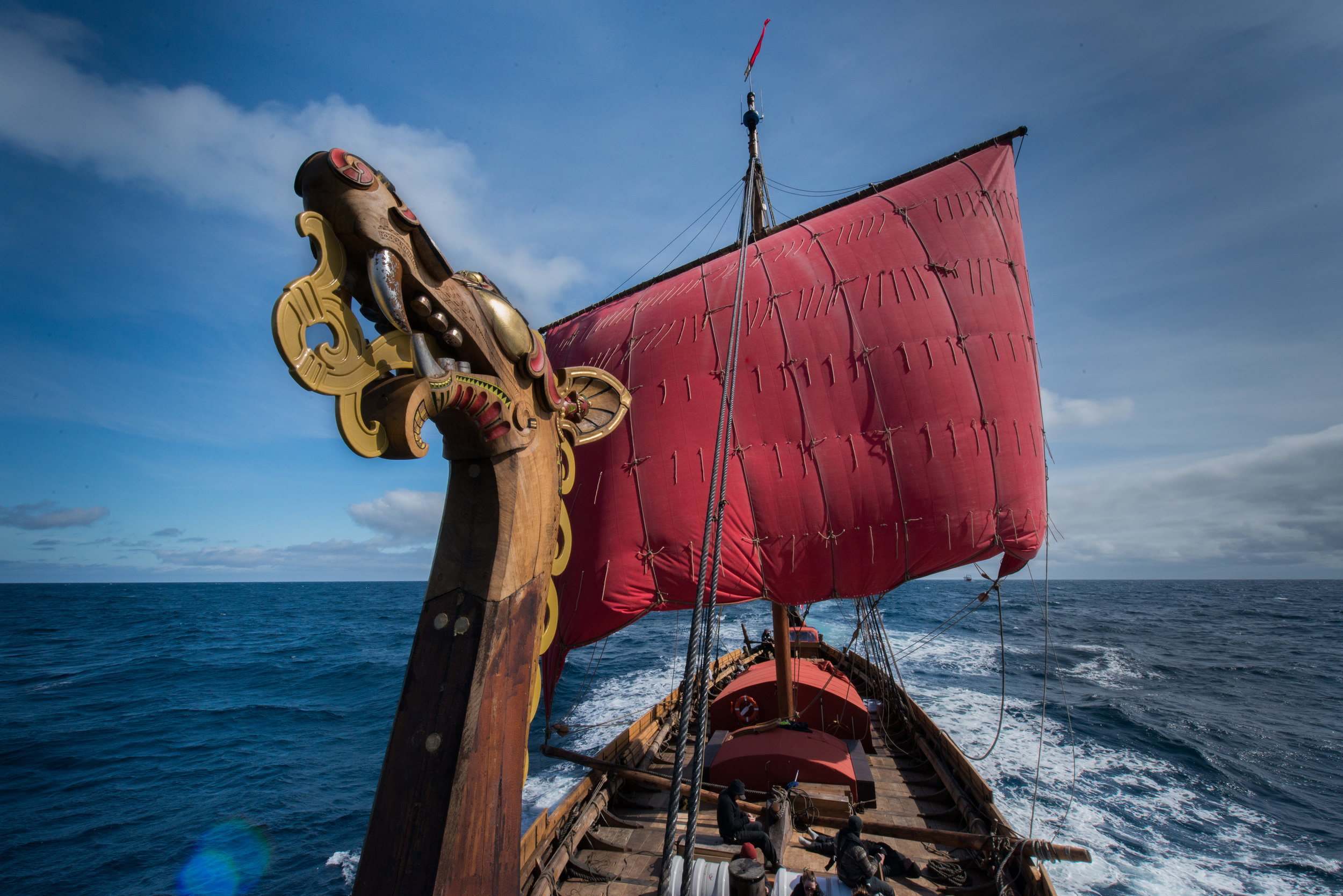This outdoor photograph captures a stunning scene on the ocean under a serene blue sky dotted with white clouds. Dominating the image is a beautifully preserved, old wooden sailboat. At the front of the boat, a meticulously hand-carved dragon figurehead rises impressively, its neck arched and fangs visible, evoking an ancient and mythical charm. The boat features a single, vibrant red sail, billowing gracefully in the wind. The detailed craftsmanship and the golden-brown tones of the dragon add a touch of grandeur. While the boat appears empty at first glance, faint silhouettes of one or two people can be seen on the deck, adding an element of mystery. The horizon shows more clouds scattered along the shoreline, enhancing the timeless feel of the scene.